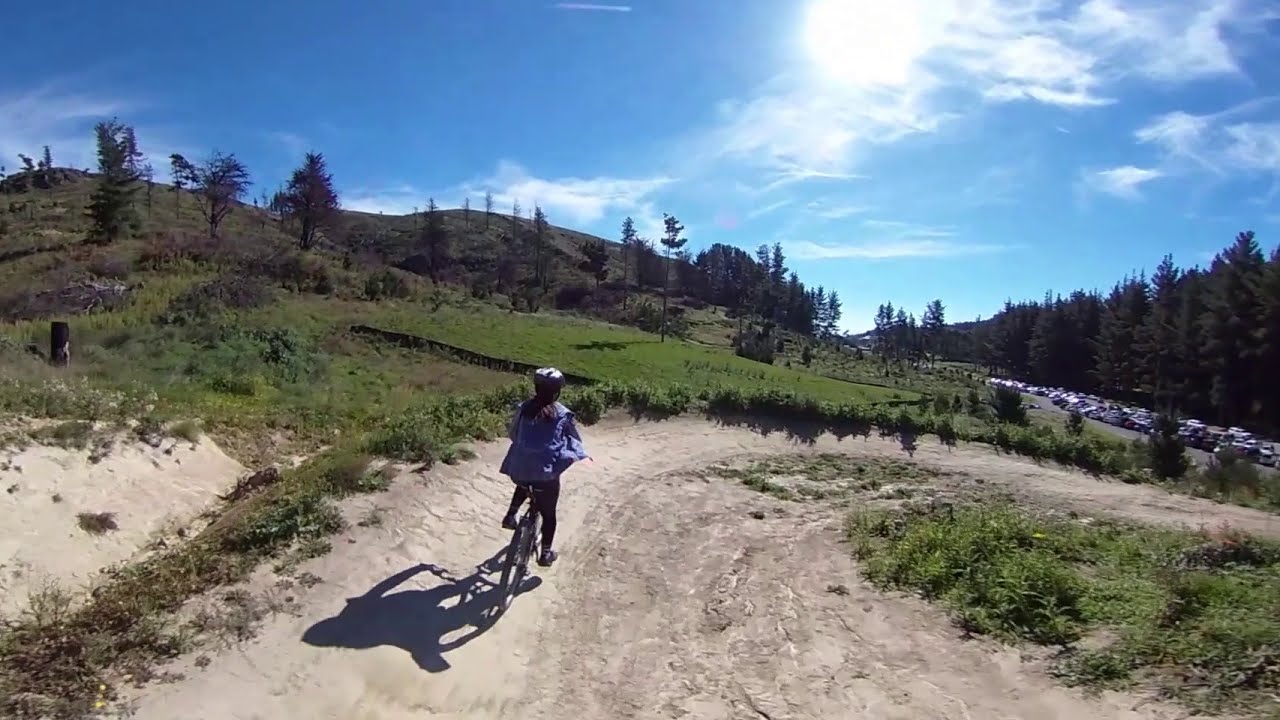The photograph captures a stunning mountainside scenery under a clear blue sky with whispers of white clouds. Dominating the image is a winding dirt path, light brown or cream in color, that curves like a horseshoe down the green, grassy hillside. In the center of the image, a woman wearing a blue jacket, black pants, and a blue helmet is seen riding her bicycle down this path. Shadows of the woman and bike trail behind her. On the left side of the path, sparse trees and patches of green grass can be seen, while the right side features more grass and smaller trees. At the bottom of the hill, a parking lot crowded with numerous cars is bordered by a dense line of trees. The overall scenery is completed by the lightly forested mountain environment, punctuated by tree stumps and illuminated by the sun high in the sky. The tranquility and beauty of the landscape add an adventurous yet serene touch to the scene.